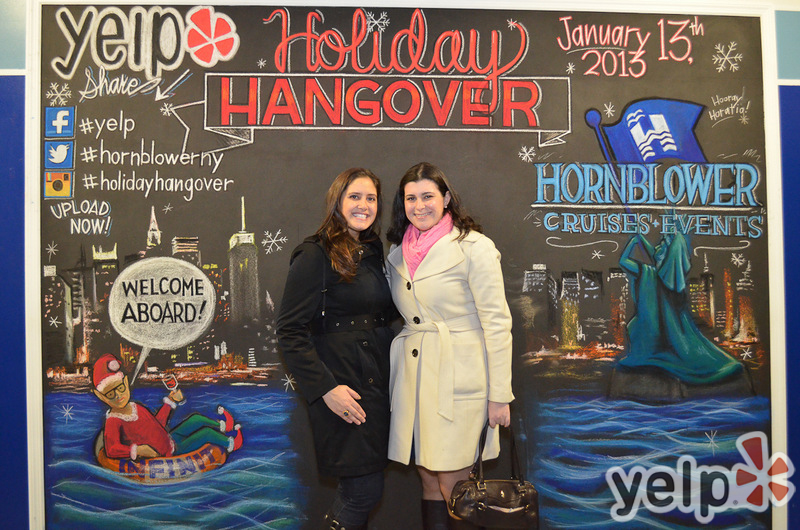Two women, appearing to be in their mid-20s with brown hair, are standing and posing for a photo in front of a large holiday-themed poster. The woman on the left is dressed in a dark gray or black overcoat with buttons around the waist and blue pants, while the woman on the right is wearing a white waistcoat adorned with three large black buttons and tassels tied around her waist. She accessorizes with a pink scarf, a large leather purse in her left hand, and boots. Both women are smiling and facing the camera.

The background poster features a New York City skyline viewed from a bay of water, depicted as a nighttime scene with a Christmas theme. The text "Holiday Hangover" is prominently displayed in red font at the top center of the poster. To the left, the poster reads "Yelp Shake" along with various social media icons and hashtags, while to the right, it says "Hornblower Cruises and Events" in blue font and "January 13, 2013." Another notable detail includes an elf floating on an inner tube in the water, accompanied by a speech bubble saying "Welcome Aboard." The overall design gives a festive and busy impression, with numerous labels and graphics.